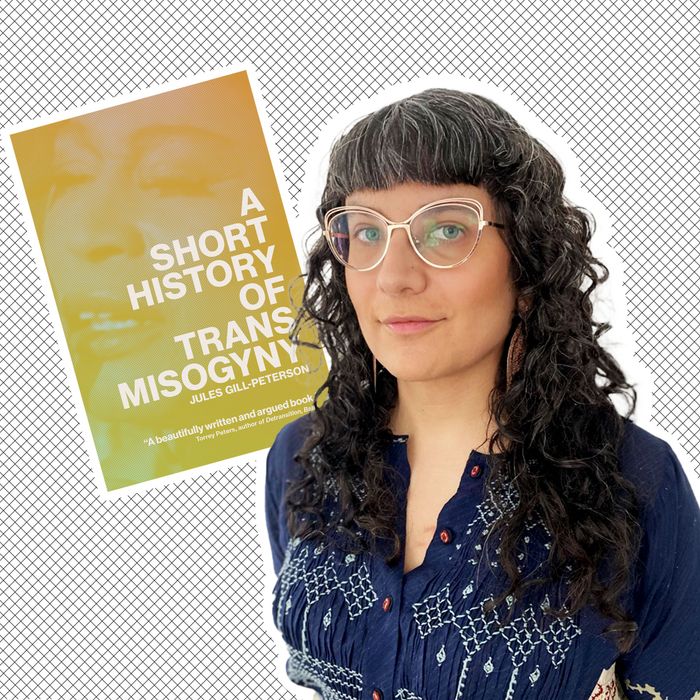This vertical rectangular image features a person standing against a mesh background composed of perpendicular lines forming boxes. The individual, who has long black hair with bangs, is wearing a textured blue blouse adorned with white stitching, triangles, and diamond shapes, and fastened with small red buttons. They are sporting large gold-rimmed glasses and pink lipstick, and their blue eyes gaze directly into the camera.

To the left of the person, above their shoulder, is a book with a gold cover and white lettering that reads "A Short History of Trans Misogyny" by Jules Gill-Peterson. Below the title, there is additional text, including a partial quote that praises the book as "a beautifully written and argued book." The overall image suggests that this person might be the author of the book.